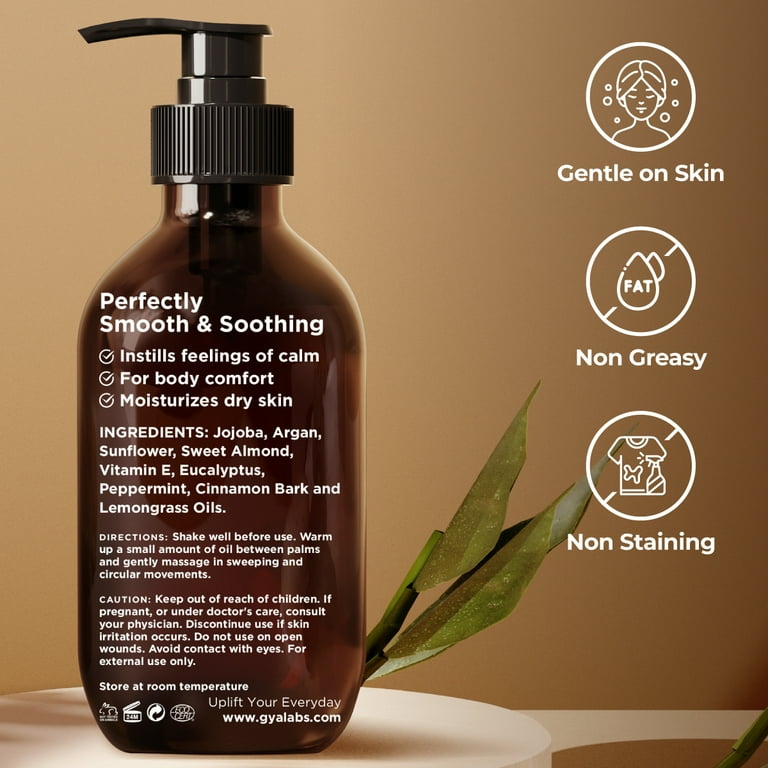This square-shaped image, approximately six inches on each side, appears to be an advertisement for a skincare product. The background transitions from a lighter brown on the left to a darker shade on the right. In the foreground, there's a dark brown glass bottle with a black pump cap, labeled with white text. The bottle features the following details: "Perfectly smooth and soothing," "Instills feelings of calm for body comfort," and "Moisturizes dry skin." The listed ingredients include jojoba, argan, sunflower, sweet almond, vitamin E, eucalyptus, peppermint, cinnamon bark, and lemongrass oils. Directions instruct users to shake well before use, warm a small amount of oil between palms, and gently massage in sweeping and circular motions. There are cautionary notes to keep the product out of reach of children, avoid use if pregnant or under a doctor’s care without consulting a physician, discontinue use if skin irritation occurs, avoid contact with eyes, do not use on open wounds, and to store at room temperature. 

To the right of the bottle, there are three white circles with icons and descriptions: one showing a person’s face labeled "Gentle on skin," another with a crossed-out fat droplet indicating "Non-greasy," and the last featuring a t-shirt and a spray bottle symbolizing "Non-staining." The bottle is surrounded by two green leaves at its base, and the web address www.gyalabs.com is featured. The image is well-lit from the left side, enhancing the text and details on the dark bottle.